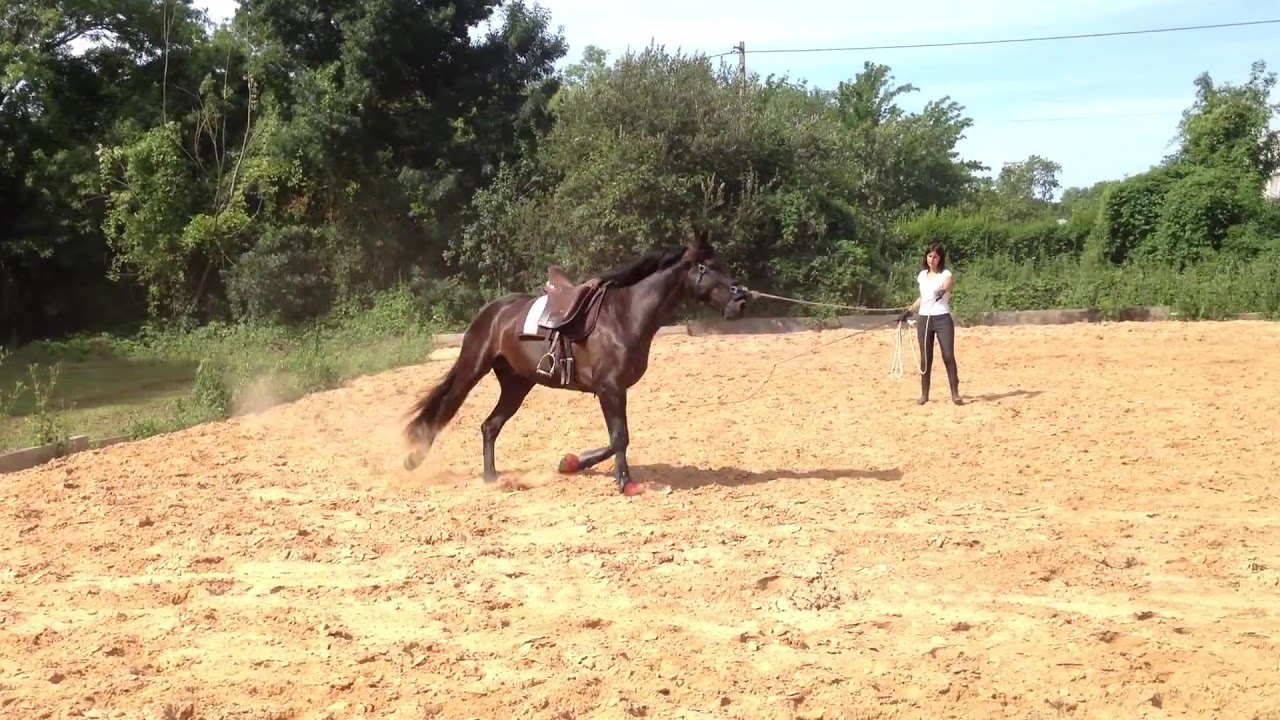In this outdoor image, a woman with shoulder-length dark hair is seen in the center of a sandy patch, holding the lead of a dark chocolate brown horse with a very dark mane and tail. The woman, dressed in a white shirt, black pants, black boots, and black gloves, stands slightly back and to the right as the saddled horse trots around her. They are surrounded by lush greenery, including bushes, vines, and various trees. Behind them, a dense forest area is visible with an oak block and power lines stretching across the upper right part of the image. The sky is blue with some clouds, adding to the tranquil, natural setting.